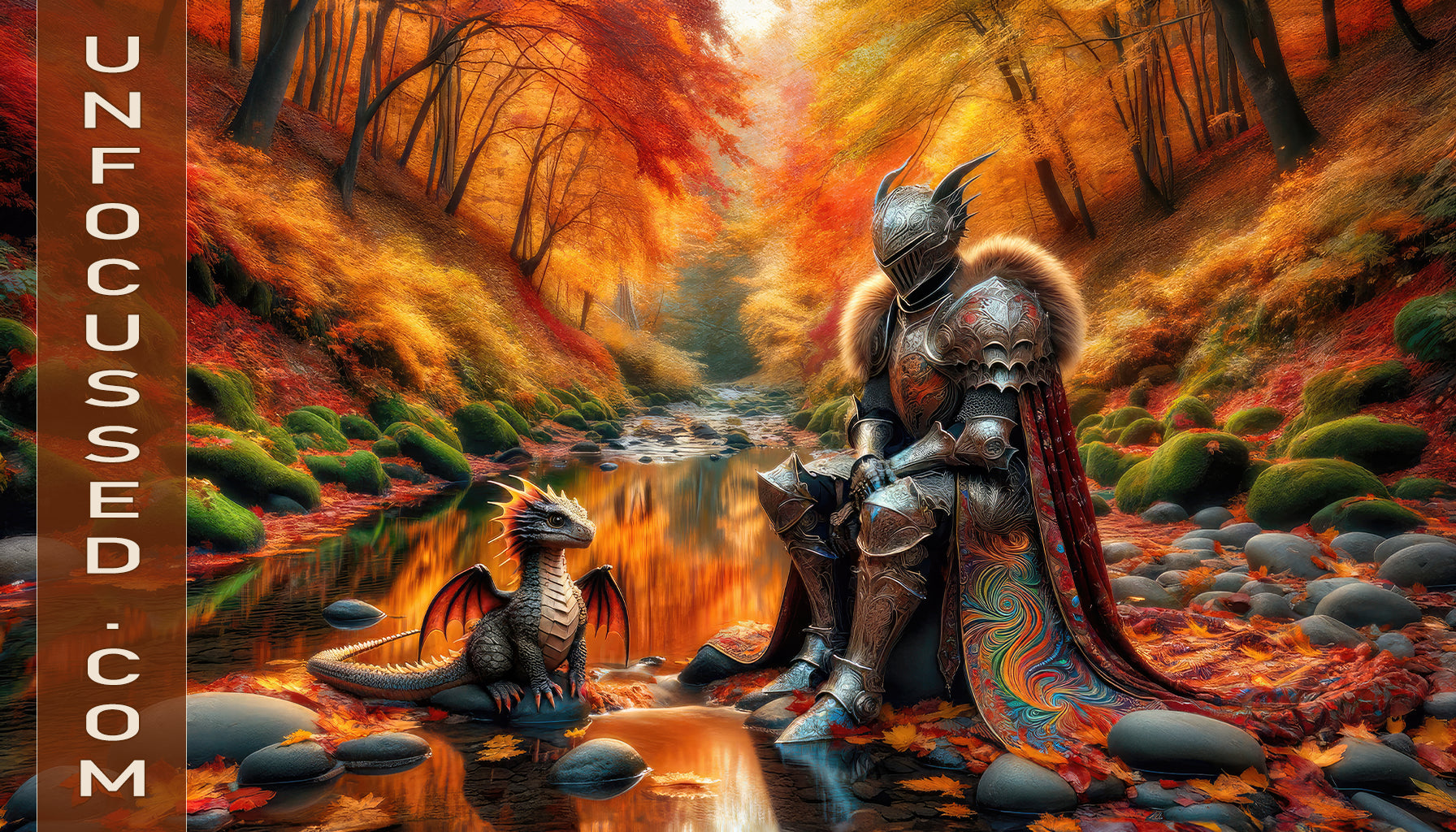The digital artwork showcases an intricately detailed knight seated confidently amidst a serene landscape, perfect for a website display. The knight is fully armored, enveloped in dark silver armor, including a helmet adorned with backward-pointing wings and a thin sliver eye mask. Massive, triple-layered shoulder shields in silver and brown, along with a fuzzy brown item featuring long, light-edged hairs on the left shoulder, contribute to his imposing presence. His metal gloves rest on his armored knees, which are heavily protected by thick knee pads. 

Within the scene, a small dragon-like creature, perched on a rock to the bottom left, adds an element of fantasy. This diminutive creature boasts wings with red and black accents, a gray-scaled body, yellow-talon feet, and a long gray tail with yellow spikes. It gazes to the right, appearing inquisitive. Both the knight and the dragon are situated in a small valley enclosed by two hills, with a tranquil, ripple-free body of water behind them reflecting orange and yellow hues. Perfectly round gray rocks scattered around are fringed with dark green moss, blending into the vibrantly colored grass hills adorned in yellow, bright red, and dotted with fall foliage trees displaying dark red, yellow, orange leaves, and black trunks.

A striking cloak with rainbow swirls of bronze, gold, green, and blue cascades from the knight's back, adding to the surreal beauty of the illustration. To the far left side, a vertical banner reads unfocused.com in white text, adding a modern touch to this enchanting and beautifully framed scene.